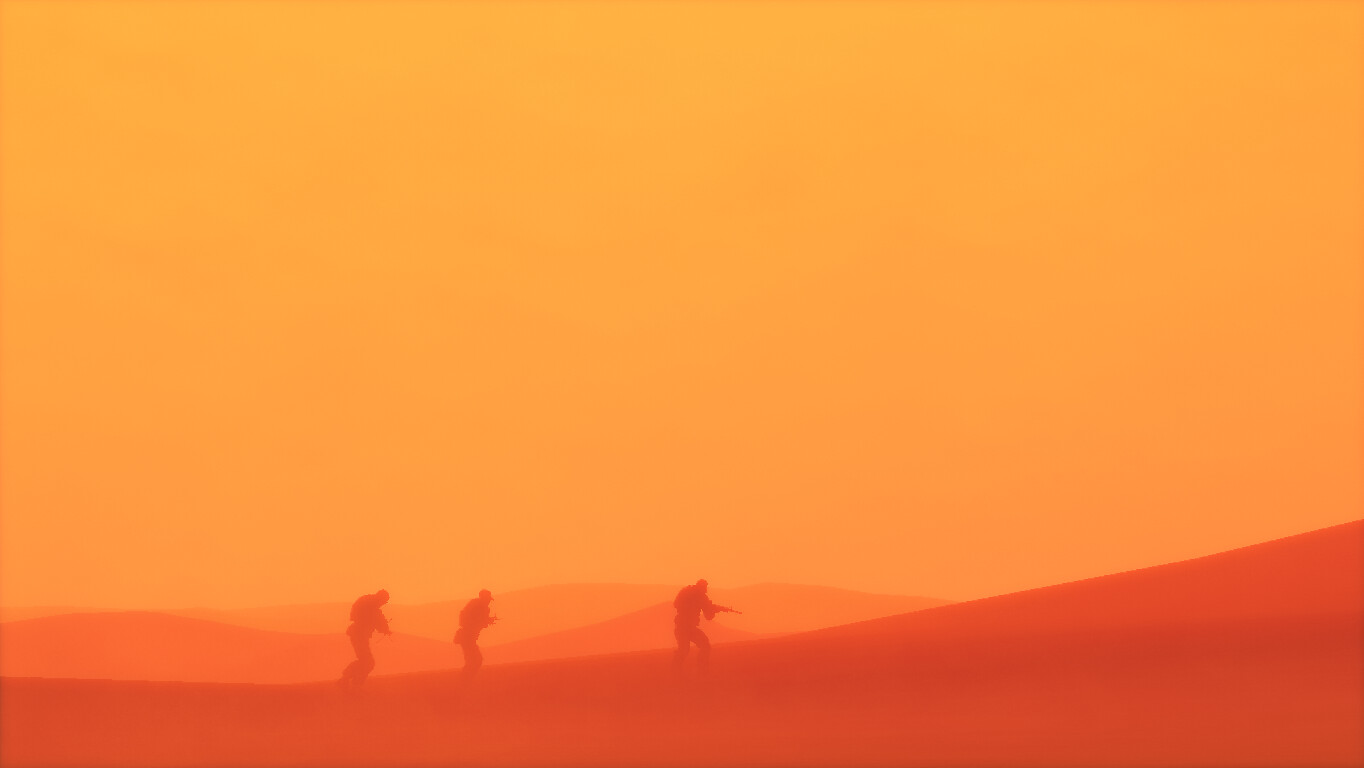This striking landscape photograph, likely enhanced with special filters, captures a vivid desert scene dominated by a golden-orange sky that occupies nearly nine-tenths of the image. The sky's rich, yellow-gold hue forms a dramatic backdrop to three men, dressed in military gear and silhouetted in dark orange. They are positioned in the lower center and are traversing an orange-hued slope that ascends from the left to the right of the frame. The foreground features a prominent dark orange hill, while behind the silhouettes, three layers of hills progressively lighten from dark orange to a paler gold shade. The men, one with a weapon drawn, move toward the right, their dark figures blending seamlessly into the tonal gradations of the desert landscape. The entire scene, with its meticulous use of varied orange tones, exemplifies artistic photographic representationalism enhanced by digital filters, creating a captivating and visually harmonious composition.